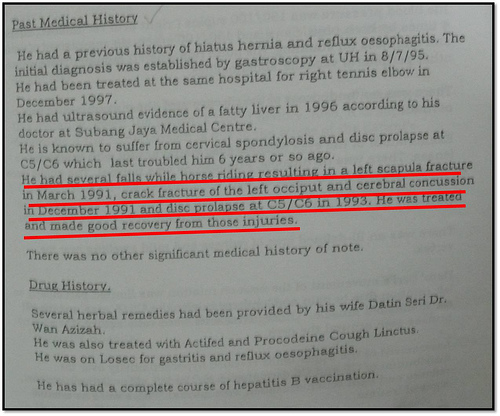The image depicts a meticulously detailed medical record of a patient, formatted within a small rectangle measuring approximately four inches wide and three inches tall, with a thin black outline. The background is gray, and the text begins from the upper left-hand corner. The title "Past Medical History" is prominently underlined. The initial entry details a history of hiatus hernia and reflux oesophagitis, diagnosed via gastroscopy at UHN on 8-7-95. Notable subsequent medical entries include treatments for right tennis elbow in December 1997, and ultrasound evidence of a fatty liver in 1996. Further complications include cervical spondylosis and disc prolapse at C5/C6, last troublesome around six years prior, as diagnosed by a doctor from Subang Jaya Medical Center. 

Highlighted in bright red underlined text, the record chronicles several falls from horse riding: a left scapula fracture in March 1991, a crack fracture of the left occiput and cerebral concussion in December 1991, and another instance of disc prolapse at C5/C6 in 1993, from all of which the patient recovered well. Subsequent to these significant injuries, the document notes no other notable medical history.

The following section, titled "Drug History" and also underlined, lists various treatments and medications the patient has received: several herbal remedies provided by his wife, Datenseri Dr. Juan Aziza, and treatments including Actifed, Crocodine Cough Linctus, and Losec for gastritis and reflux oesophagitis. It further notes the patient has completed a full course of Hepatitis B vaccination.